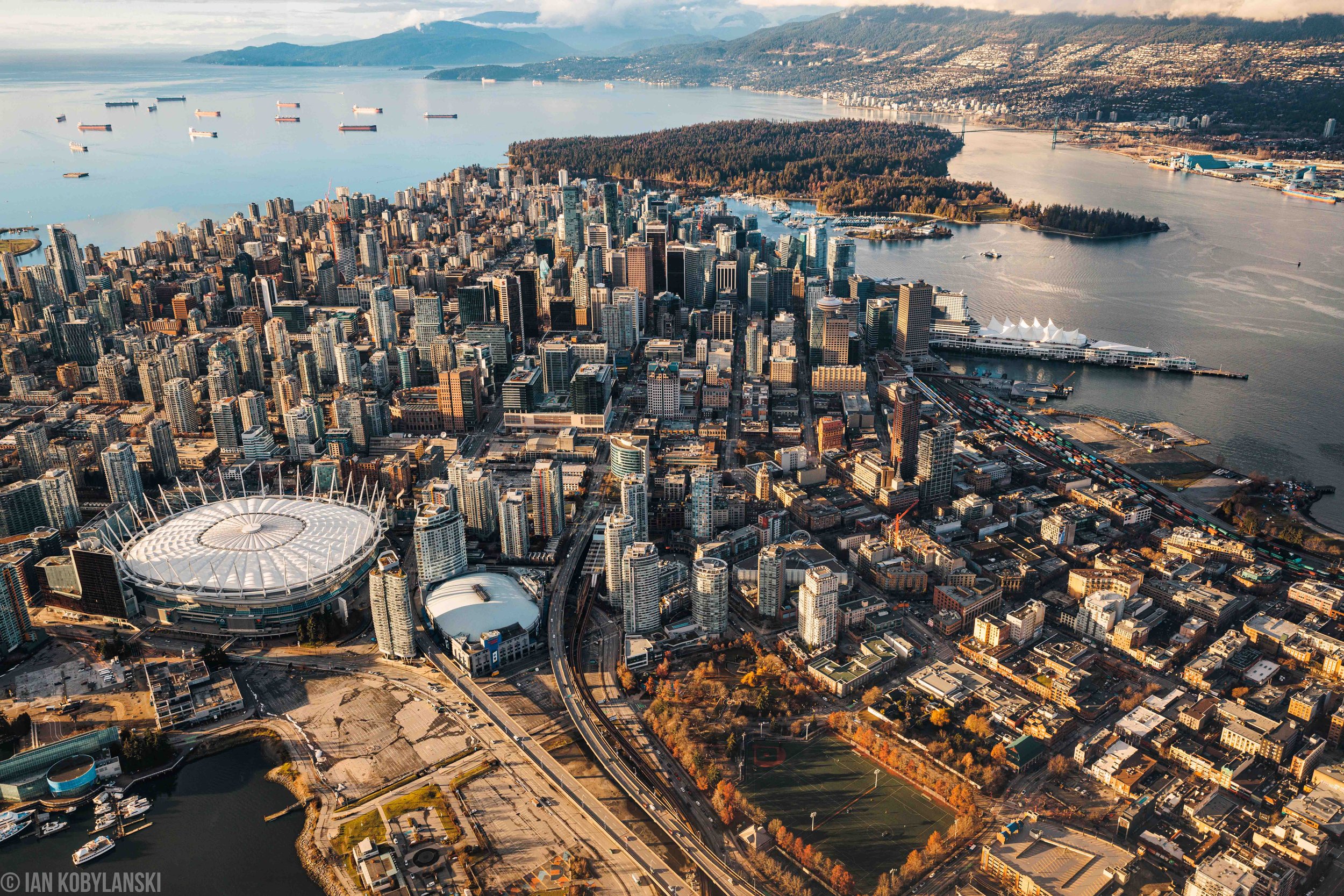This vibrant aerial photograph, likely taken from a drone or helicopter, provides a stunning top-down view of Sydney, Australia, showcasing a bustling metropolis nestled along a vast body of water. Dominating the image are numerous towering skyscrapers scattered throughout the densely populated cityscape. Towards the bottom left of the image, a prominent feature is the distinctive Sydney Opera House, while nearby, a large sports dome - possibly a stadium - further underscores the city's architectural wonders. A notable freeway cuts through the city landscape, weaving from the bottom towards the sports dome and beyond.

In the foreground, a soccer pitch, surrounded by autumn-hued trees, adds a splash of earthy colors to the urban setting. To the left, amidst the cityscape, some areas are under construction. The bottom-left corner reveals a pier, with boats moored nearby, contributing to the city’s status as a significant port city. On the top right and top left, the water body, possibly a lake or part of the sea, is dotted with cargo ships and features several piers. Vacation homes and amenities are visible along these piers, hinting at recreational activities. An island, lush with woods and trees, sits just off the coast, accessible by boats, adding a natural element to the urban environment. The photograph is credited with a copyright to IANKOBYLANSKI, indicating its professional composition and ownership.